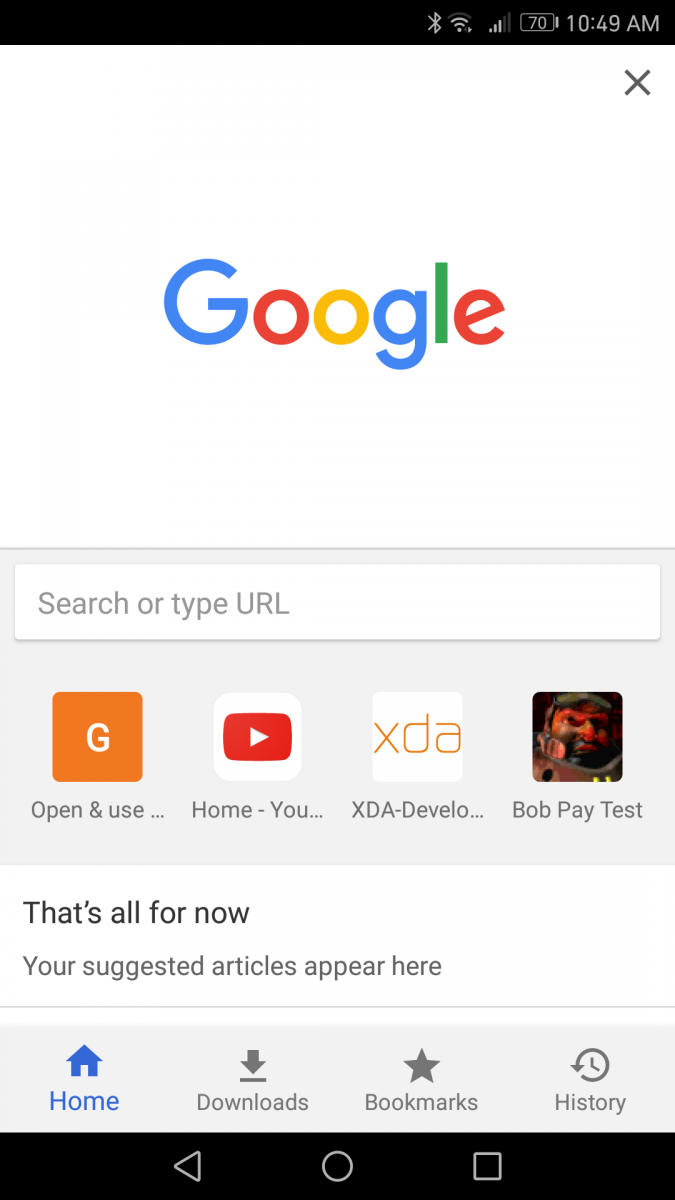In this screenshot taken from a smartphone at 10:49 a.m. with a 70% battery level, the screen displays a predominantly white background featuring the Google homepage. The familiar Google logo, composed of letters in blue, red, yellow, and green, is prominently placed at the top. Below the logo, the text "search or type URL" is visible in the search bar.

Further down, there are several colored icons and labels. An orange box with a white "G" inside it is labeled "open and use." Adjacent to it, a red box with a right-pointing arrow is labeled "home," and another icon beside it says "you." A white box displaying the text "XDA" represents the XDA Developers forum. Another box next to it features an image of a warrior or fighter with the text "Bob A. Test."

Following these icons, a message states, "That's all for now. Your suggested articles appear here," though no articles are currently visible on the screen. The bottom of the interface includes options labeled "home," "downloads," "bookmarks," and "history," accompanied by navigation buttons for back, home, and close at the bottom of the screen.